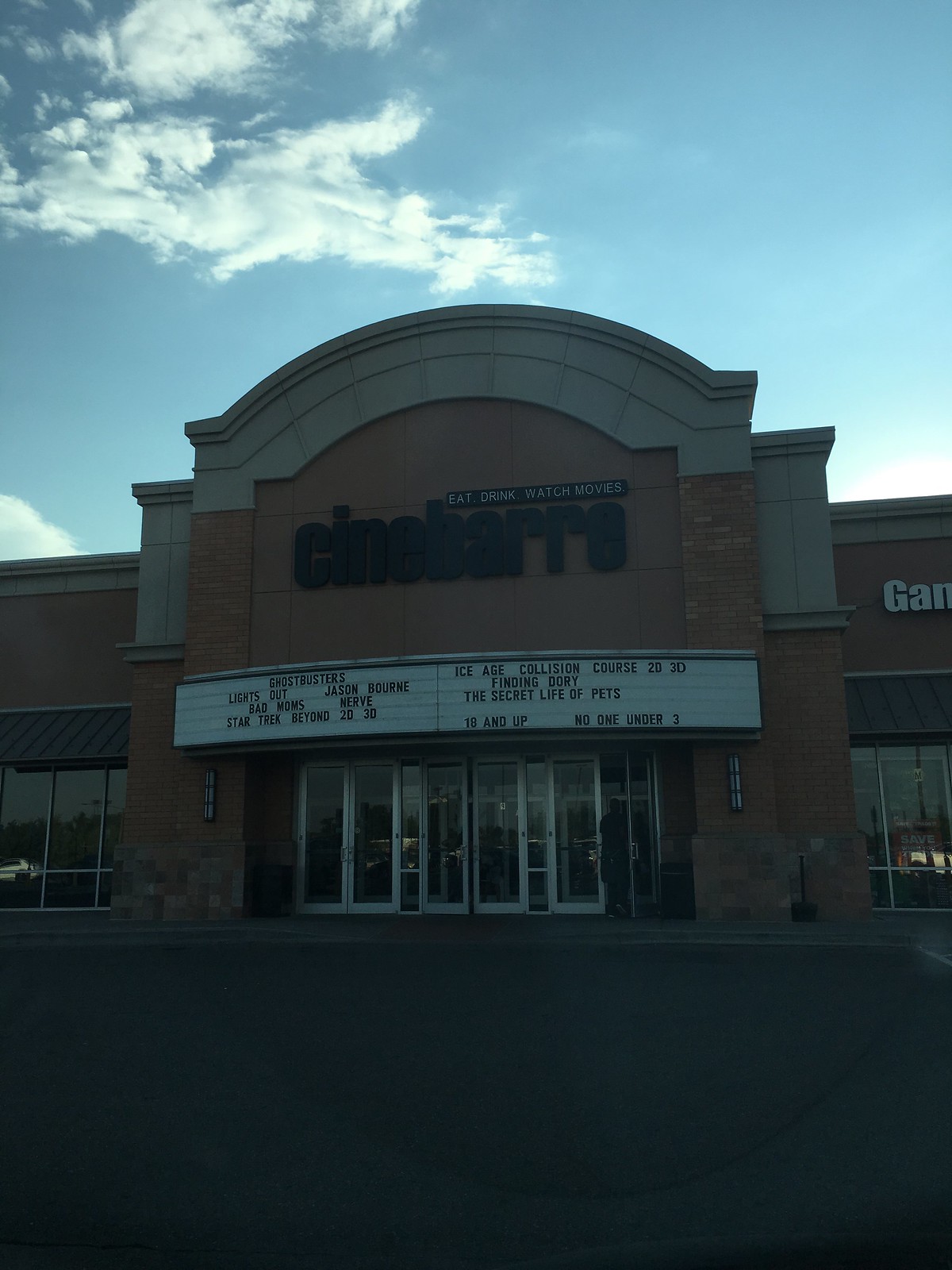This image captures the front of a C-I-N-E-B-A-R-R-E cinema located in a strip mall setting. The photo is taken from the parking lot, which occupies about a third of the foreground. The cinema is a couple of stories high, featuring three sets of silver perimeter glass doors for ample entry and exit. Above these doors, a white marquee with black lettering lists the movies currently showing: Ghostbusters, Lights Out, Bad Moms, Star Trek Beyond, Ice Age: Collision Course, Finding Dory, and The Secret Life of Pets. The cinema's large, rounded-top façade displays the words "CINEBARRE" prominently, accompanied by the tagline "Eat, Drink, Watch Movies," suggesting it's a cinema bar. To the right of the cinema, a partial sign for GameStop is visible, displaying "G-A-M." On the left, another shop is present but its identity is not discernible in the image. The building appears dimly lit, likely because the sun is positioned just behind it, casting a shadow over the scene.